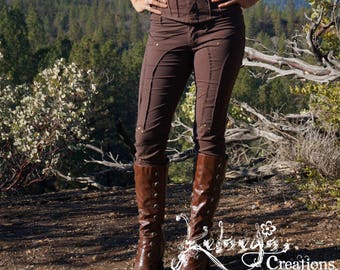This is a small, rectangular, horizontal photograph, primarily focused on a woman from the waist down, standing on a dirt trail. She is wearing tight-fitting, brown pants and knee-high leather boots in a different shade of brown. Her hands, visible at the hips, indicate she is facing the camera. The background features a good-sized boulder and some landscaping, including a bush with white flowers to the left and evergreen trees further back, blending into a dark green coniferous forest. The image includes a signature in flowy script at the bottom right corner, with "Kelsey's Creations" indicated clearly beneath.